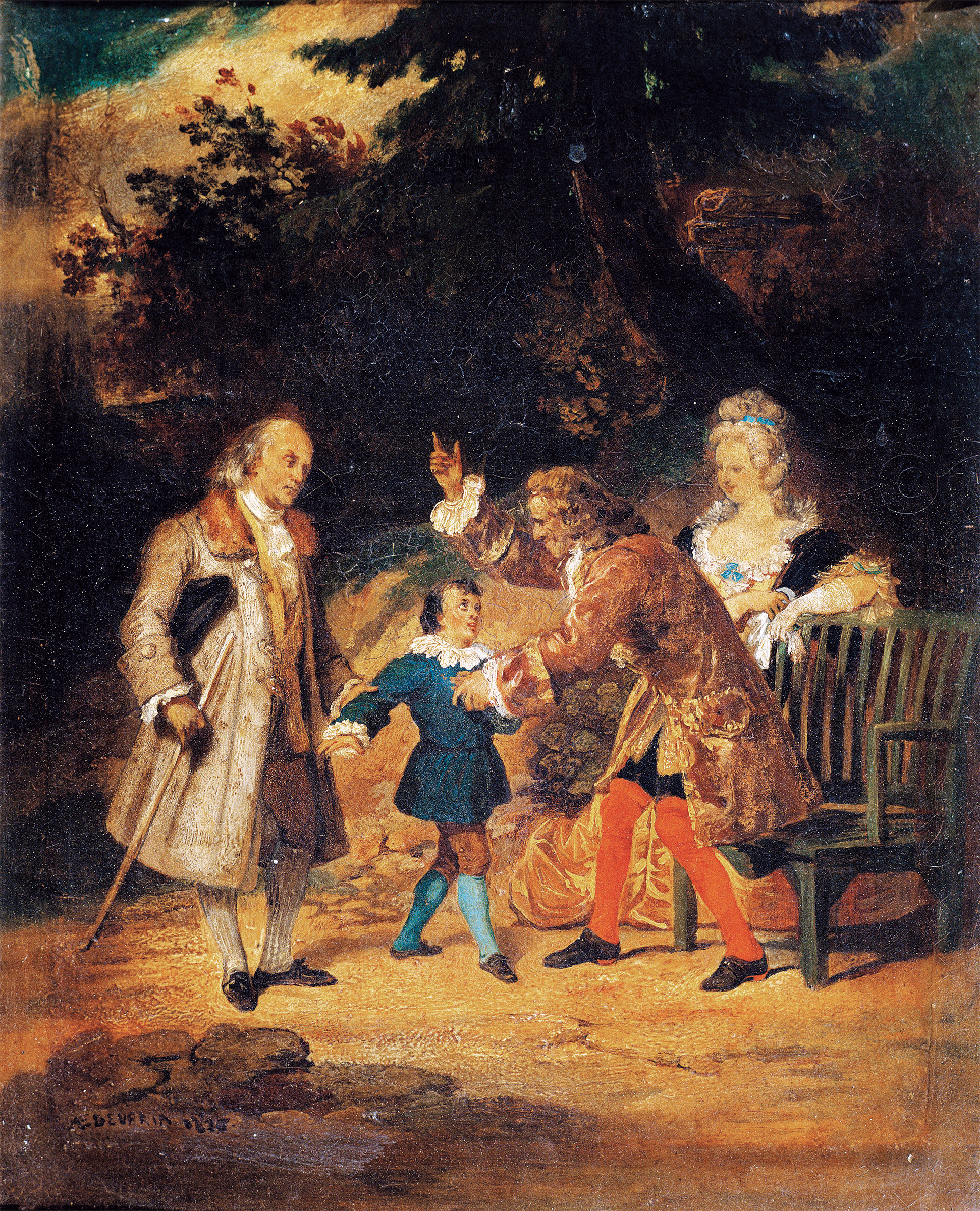The oil painting, dating back to the 18th or early 19th century, depicts an elaborate outdoor scene with four figures dressed in period attire. On the left, a distinguished elderly man resembling Benjamin Franklin or George Washington holds a hat under one arm and a cane in the other, while clasping the wrist of a young boy. The boy, ambiguously dressed in a blue smock, high blue socks, and a fluffy white collar, gazes upwards with an expression of concern or curiosity. Next to the boy is another man in a long brown coat and striking red stockings, his hand raised as if in reprimand. Completing the scene is a seated woman with her hair styled in an elaborate updo, dressed in an elegant gown and white gloves, positioned on a bench in the foreground. The background is dark and atmospheric, possibly indicating nightfall, with a prominent tree featuring thick green foliage, through which a sliver of light sneaks in from the upper left corner. The painting's aged appearance, marked by cracks and imperfections, enhances its historical authenticity and depth.